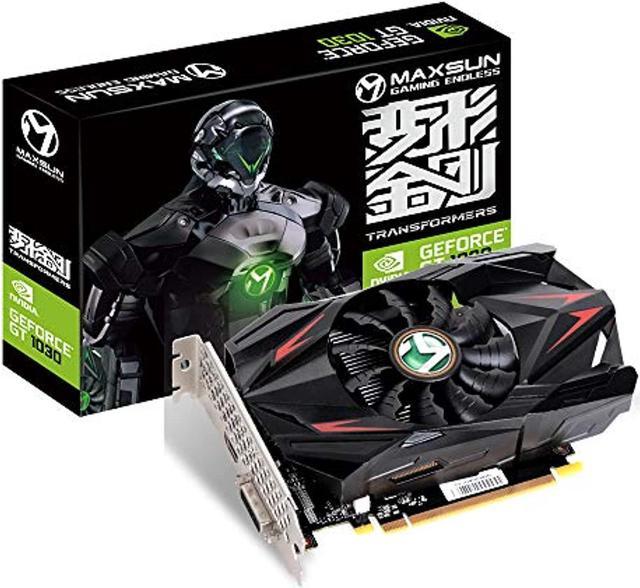This image showcases a high-end graphics card, specifically the MaxSun Gaming Endless Transformers GeForce GT 1030. The card itself has a distinct, stylized design reminiscent of a sports car, featuring sharp angles, a large black fan with a green center bearing a white "M" logo, and sleek black and red accents. The packaging is predominantly black and displays a 3D-rendered image of a warrior in black and silver mechanical armor, also bearing the "M" logo. The overall presentation and details emphasize the card's advanced capabilities and suitability for high-powered gaming computers.